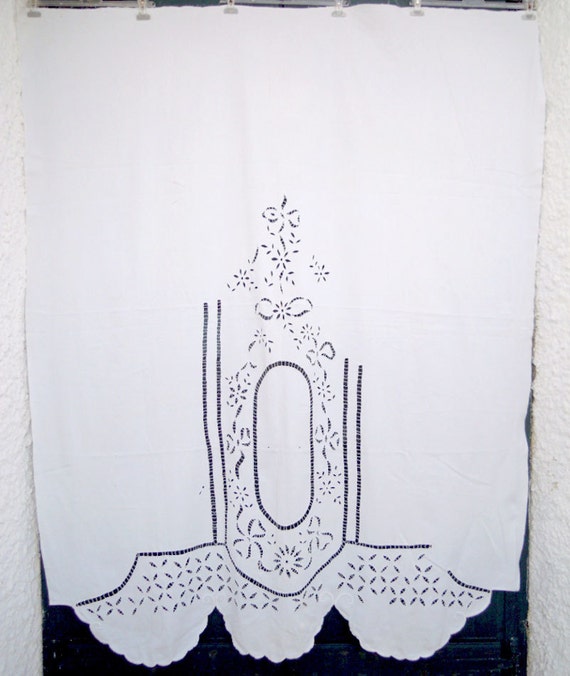This color photograph captures a detailed image of a white curtain hanging in front of a window framed by white textured stucco walls. The curtain, held in place by six plastic hooks attached to a curtain rod, features intricate lace embroidery. Dominating the textile are a tall floral design and cutout lace bows, which extend nearly to the top. The bottom edge of the curtain is scalloped into three distinct panels, with an array of lace X's embellishing it. The curtain almost entirely obscures the window, which has a dark wooden or black metal trim, and the small visible area at the bottom indicates it is night outside.